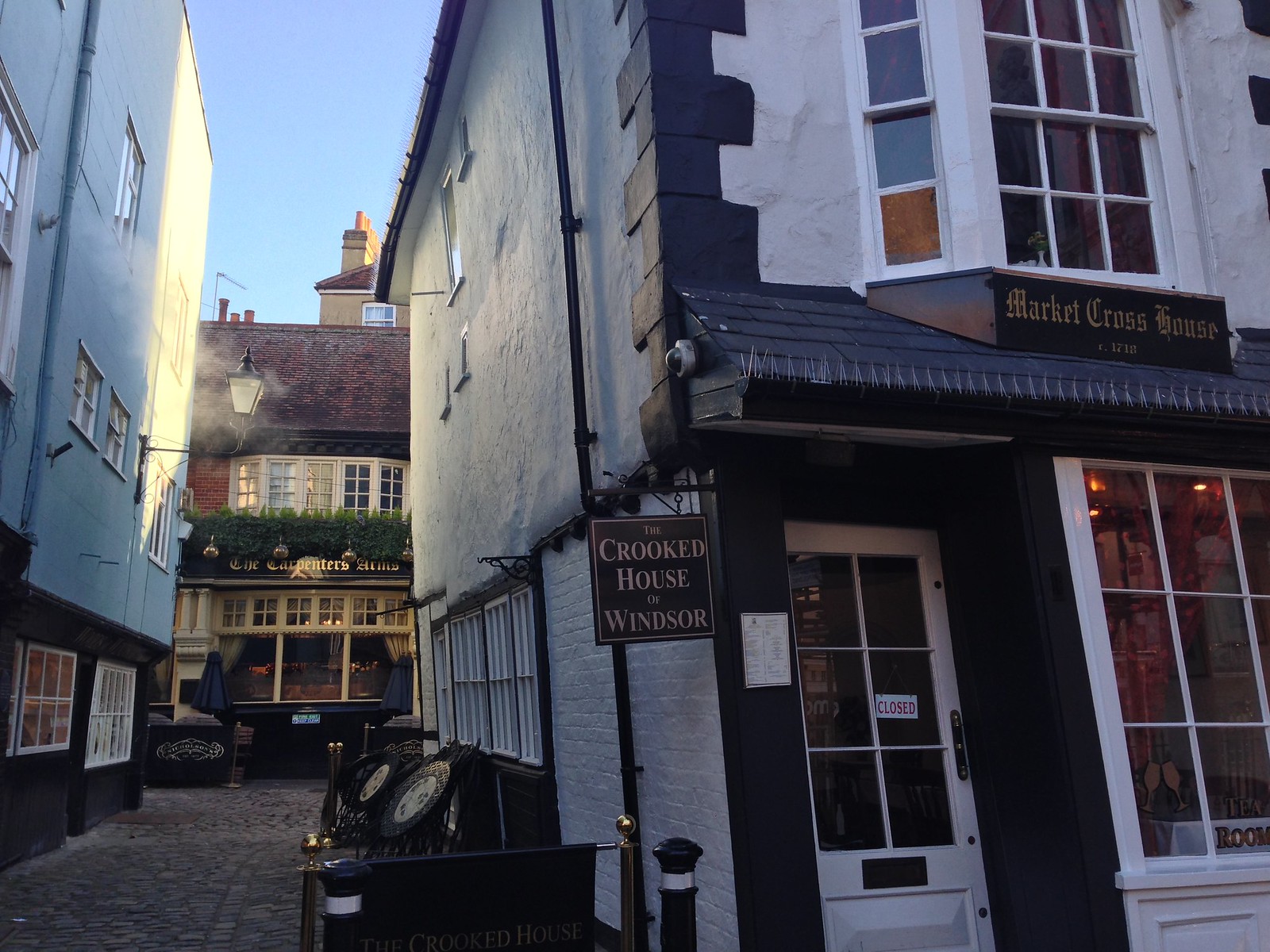The image showcases an outdoor view in a quaint city center, centered around the historical Market Cross House from 1718. The scene is dominated by a two-story building on the right, which features a white facade with black brickwork edges and a sign that reads "Market Cross House." Below this, there is an awning and a white door marked "Closed." Adjacent to the door hangs a sign that says "The Crooked House of Windsor," a name emphasizing the unique architectural style of the structure.

Positioned to the left of the main building is a narrow street lined with folded tables. The street separates Market Cross House from another white building with a black base and white-framed windows. In the distance, across this alley, stands The Carpenter's Arms, an old-style building with yellow pillars and a thatched brick roof. Green vegetation adorns a terrace above the entrance. This background building adds layers of historical and architectural interest with its ornate features and shut umbrellas in front.

The scene is brightened by the blue sky visible between the buildings, while the ground is paved in gray. Various details, including plants, signs, and an old lantern window, contribute to the bustling yet historical atmosphere of this charming city center.